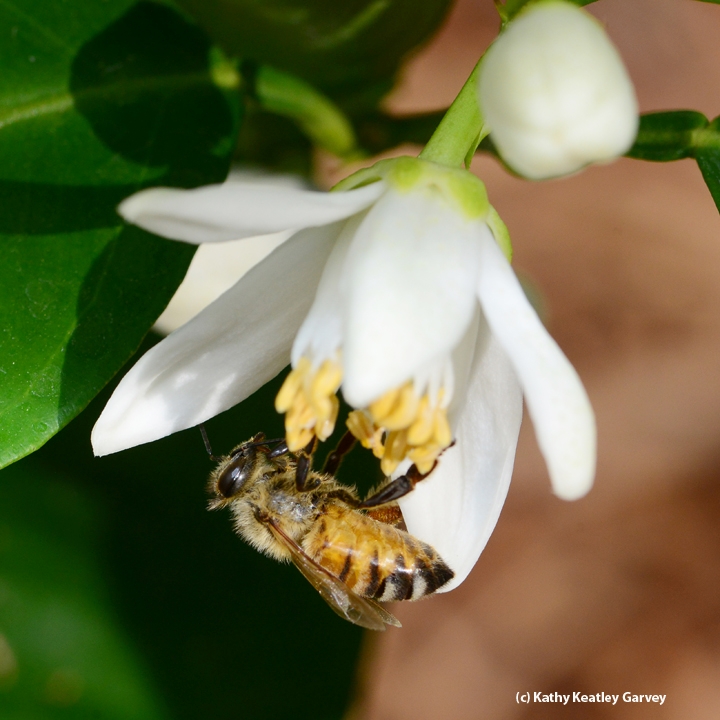The image features a detailed close-up of a bumblebee diligently pollinating a white flower, which resembles the Bells of St. Mary or a white jasmine flower. The bloom hangs downwards from a light green stem, with its petals creating a delicate frame around the yellow stamens. To the top right, a bud still waiting to bloom is visible. The bumblebee, upside down, is perched on the yellow parts of the flower's stamens, with its fuzzy torso and large head clearly observed. The creature's body showcases a striking pattern of yellow and black, common to bumblebees. Bright green leaves dominate the left side of the background, while the right side fades into an out-of-focus brown. Adding a professional touch, the bottom right corner of the image bears the watermark of photographer Kathy Keatley Garvey.